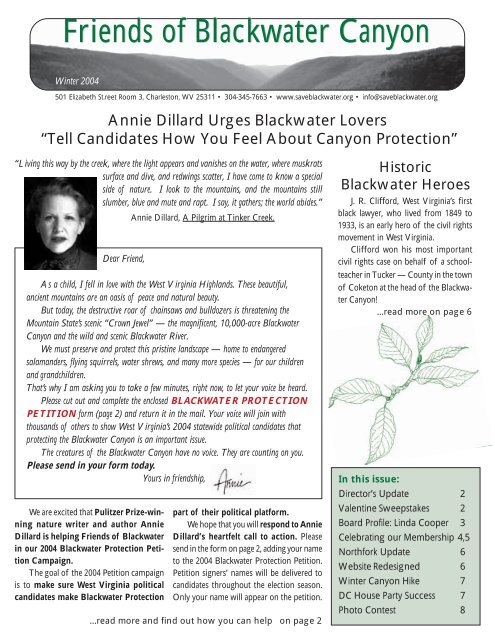The vertically aligned rectangular image presents a detailed page primarily featuring text and a few illustrations. At the very top, the header "Friends of Blackwater Canyon" is displayed prominently in green letters. Directly below the header, there is a black and white illustration of a canyon landscape. The lower left of this section is marked with the caption "Winter 2004."

Beneath the canyon illustration, a heading reads, "Annie Dillard urges Blackwater lovers: 'Tell candidates how you feel about canyon protection.'" Directly below this, a small black and white photograph of a woman, identified as Annie Dillard, is shown. She has short dark hair and is wearing a dark-colored shirt. Adjacent to her image is a quote from her book "Living by the Creek."

Following the quote, there is a boxed letter from Annie Dillard addressed to "Dear Friend." The letter emphasizes the importance of protecting the Blackwater Canyon and calls for action from the readers. Dillard recounts her childhood love for the West Virginia Highlands and describes the current threats to the Blackwater Canyon due to industrial activities. She urges readers to sign and send in a petition to demonstrate public support for canyon protection, concluding the letter with "Yours in friendship, Annie."

To the right of this section, under the heading "Historic Blackwater Heroes," there are two paragraphs detailing the contributions of J.R. Clifford, West Virginia's first Black lawyer and a civil rights pioneer. A line drawing of leaves on a twig accompanies this text.

At the bottom right corner of the page, a green boxed section titled "In this issue" lists the contents and corresponding page numbers, such as the Director's Update, Board Profile, and various events and success stories. Additional contact information for the Friends of Blackwater Canyon, including an address, phone number, and website, is also provided.